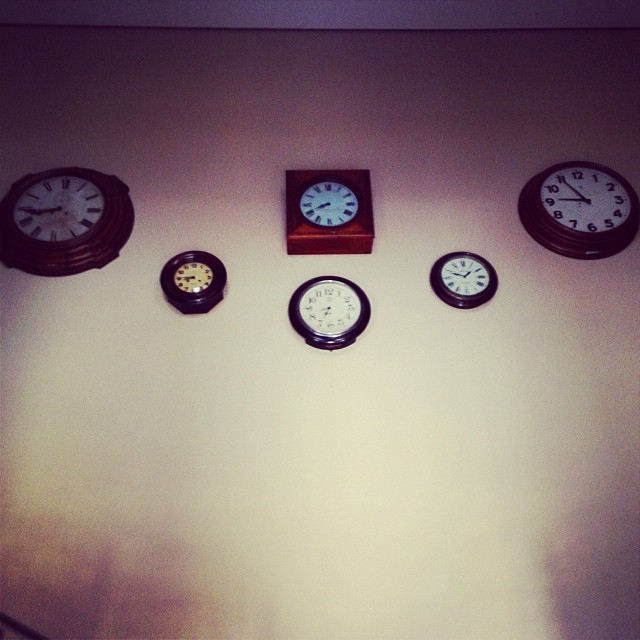This image depicts a visually striking wall adorned with an array of various clocks. They are arranged in two rows against a pristine white background, creating a decorative and intriguing display.

In the top row, the far left clock features a thick wooden case with a round face displaying elegant Roman numerals. Adjacent to it, still within this row, is a square-cased clock, also wooden and marked with Roman numerals. The third clock in this sequence mirrors the first in its round shape but diverges with standard English numerals; it reads 9:55.

The bottom row presents a more dynamic and decorative arrangement of smaller clocks. The two outer clocks in this row are positioned slightly higher than the clock in the center, creating a visually appealing staggered effect. On the left, we find a round clock with a smaller face and English numerals. The central clock boasts a dark-colored round case and faint numbers, adding to its distinctive appearance. To the right, another small clock completes this row, featuring a round dark case and Roman numerals.

This carefully arranged collection of timepieces combines various shapes, numbers, and sizes to create a harmonious yet diverse composition.